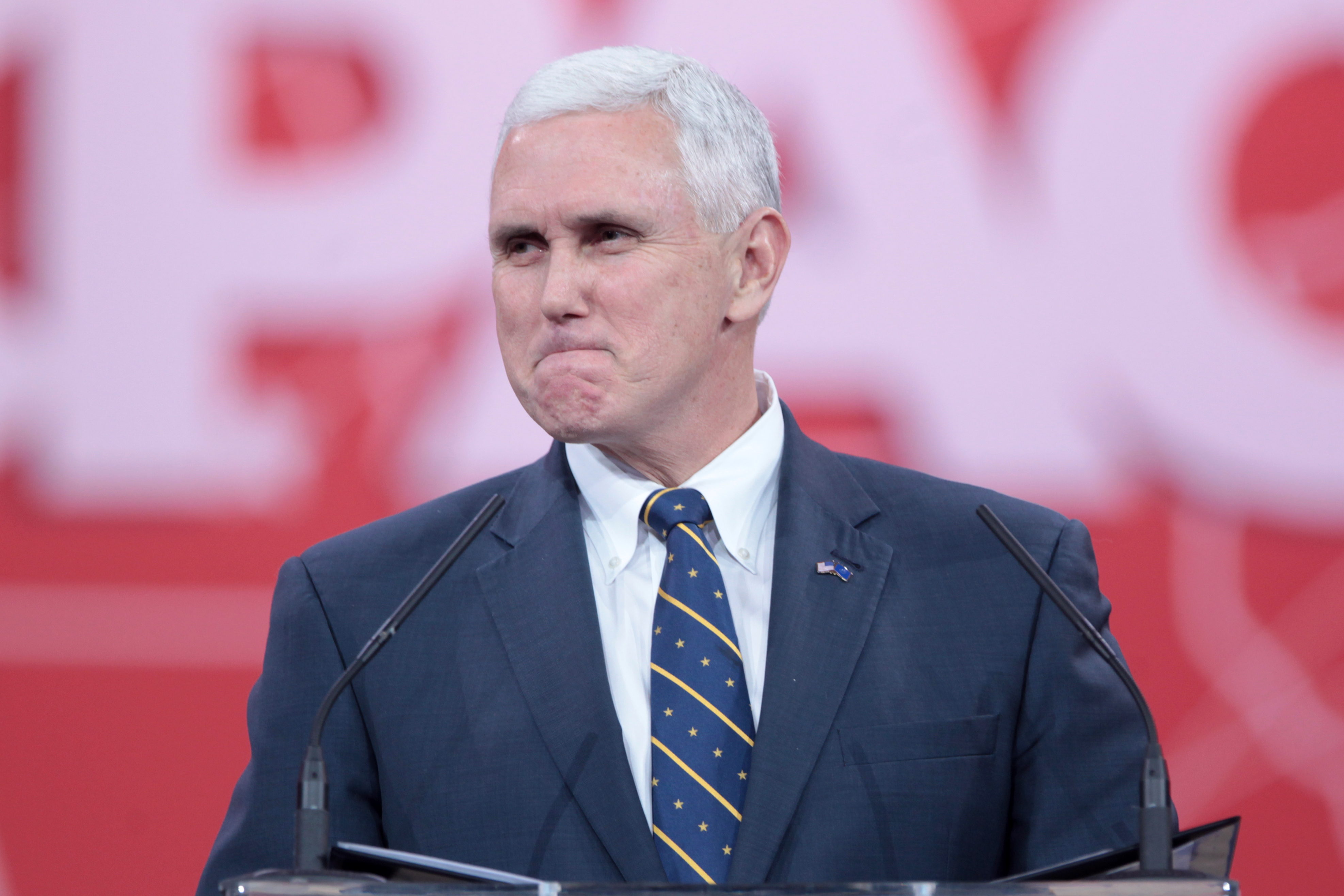In this photo, Mike Pence is captured from the chest upward, standing at a lectern or podium with two microphones angled towards him on either side. He is dressed in a dark blue suit jacket, complemented by a white shirt and a navy blue tie adorned with gold stars and stripes. A small American flag pin decorates his jacket lapel. His hair, short and white, frames his face as he gazes slightly to the left of the image. His mouth is closed with both lips pulled inward, giving a somewhat grim expression, and his chin is slightly raised. The background, which is out of focus, is red with large white letters spelling out "PAC."